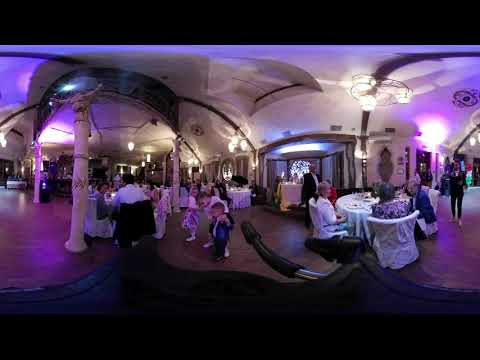The photograph captures an indoor scene at a formal gathering, likely a wedding reception or similar event, taken with a fisheye lens. This lens creates a distinctive distortion, giving the image a wavy, panoramic feel, particularly evident at the bottom and the curved walls in the background. The setting appears high-class, located in a restaurant or entertainment hall with white cylindrical columns, white walls, and a white ceiling. Round tables draped in long white tablecloths are scattered across the room, with guests elegantly dressed in suits and dresses seated at them. The high-ceilinged room is illuminated by lights above, contributing to an overall well-lit ambiance. 

In the center of the photograph, three young children—two girls in dresses and a boy in a suit—are highlighted. The floor is tiled in a dark red or brown color. On the right side, servers in black suits and white shirts are seen moving towards the tables. The image includes a thin black header and footer, suggesting it might have been taken using a smartphone attached to a selfie stick, which is slightly visible at the bottom of the picture. The overall impression is of a well-organized, elegant event captured with a unique lens that adds a bubble-like effect to the scene.